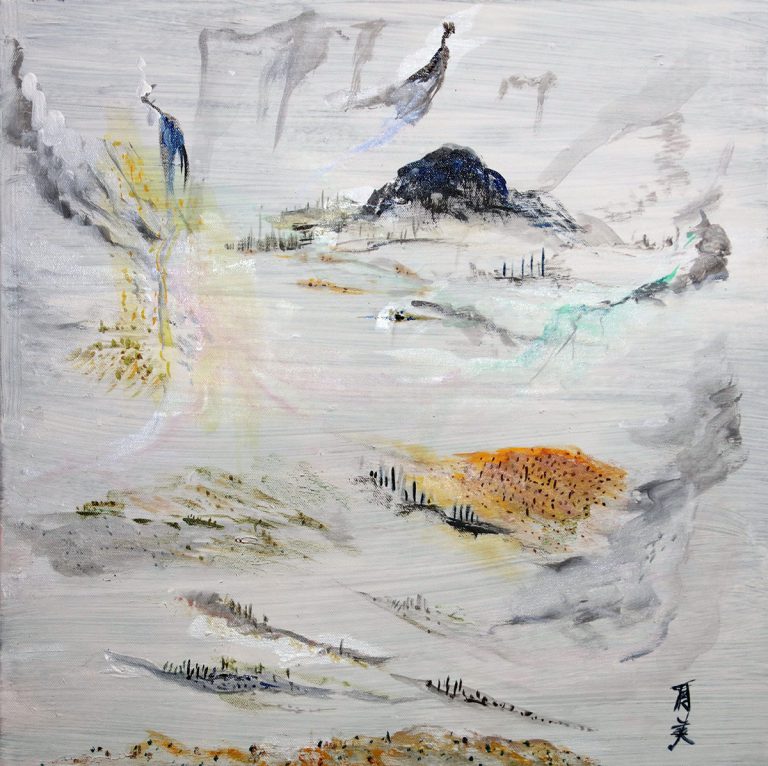This image is a photograph of a painting featuring a complex landscape depicted on a grayish background with various shades of dark and light gray. The scene includes small etched-out areas of land with diverse elements. On the left side, an animal climbs amid rising smoke, adding dynamic movement. The bottom part of the painting contains varied terrain; the bottom right is a desert area, adorned with cacti and red-brown land. Close by, Asian characters form an artistic signature, emphasizing the piece’s cultural touch. The bottom features a brownish hill that contrasts with lighter hills marked by black lines, possibly representing trees or grass. Slightly above the center, the ground shifts from white on the left to brown on the right. In the upper region, there is a cliff with glowing yellow lights, adjacent to a dark hilltop surrounded by sentry-like structures. The sky is depicted with hanging black drapes, adding a sense of foreboding. Throughout the painting, various birds, potentially peacocks, are indicated by their blue bodies and grayish long necks, though their specific details are somewhat smudged and indistinct. A dark, blue-tinted peaked mountain with grayish plants at its base is visible, alongside a yellow tree with pronounced yellow leaves.